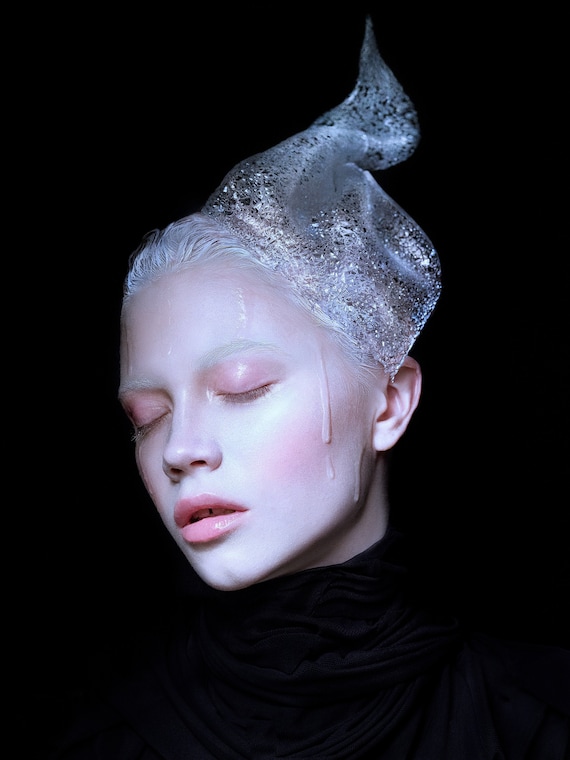The image captures a striking portrait of a figure with pale skin and ethereal blonde hair, set against a seamless black background that emphasizes their delicate features. Dressed in black clothing that appears to blend into the void, the focus is drawn to their face and head. Their eyes are closed, enhancing a serene expression, while their lips, cheeks, and eyelids are adorned with subtle rosy hues.

The hair, short and almost white, is intertwined with some kind of ornate decoration that ascends from their head in a swirling, snail-shell-like formation. This elaborate headpiece is a translucent blend, shimmering with black and silver glitter, giving it an almost icy or wax-like appearance. This aesthetic is further enhanced by the intriguing detail of what seems to be melted wax or silver goop dripping down the left side of their face and across the right eyelid.

Their eyebrows are very light, almost blending into their ghostly complexion. The person's head is slightly tilted to the left, and their face is turned slightly in the same direction, making them appear lost in a dreamlike state. This combined with the abstract headpiece and fluid elements creates a surreal and captivating visual.